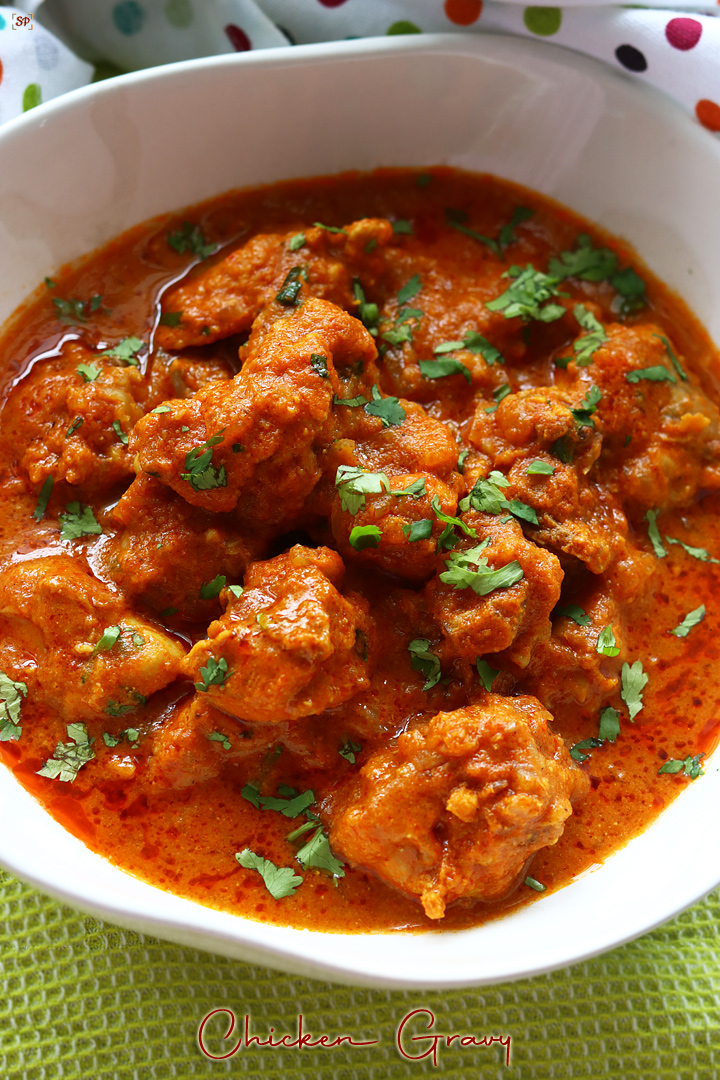This photograph features a sumptuous dish of chicken gravy, elegantly presented in a deep, white bowl. The chicken pieces are shaped into meatball-like rounds and bathed in a thick, reddish-brown sauce that hints at a rich blend of curry and possibly chili sauce, with natural oils adding to the luscious texture. Generously garnished with vibrant green parsley or cilantro flakes, the dish not only promises a burst of flavors but also pleases the eye with its contrasting colors. The bowl is artfully placed on a green waffle weave cloth, while a colorful cloth with multicolored polka dots is draped around it, adding an aesthetic touch to the presentation. The image includes a small, cursive text in red at the bottom, reading "chicken gravy," underscoring the dish's identity without the presence of any silverware, likely to focus all attention on the appetizing meal.